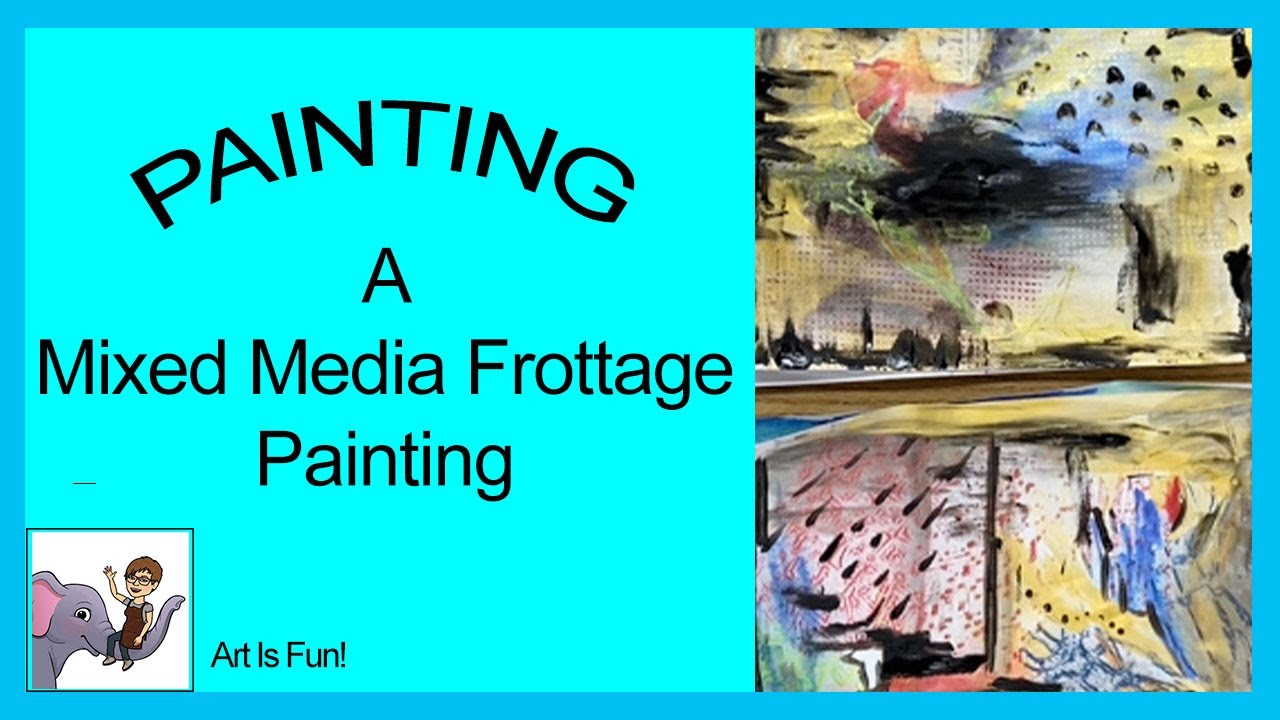The image is a horizontal, full-color print bordered by a blue frame. The left section features a green background with the title "Painting a Mixed Media Frottage Painting" in black, capitalized letters. At the bottom left, there is a small white box that contains a cartoon of a smiling elephant lifting a cheerful woman with glasses and short hair on its trunk, next to the phrase "Art is Fun" in black letters. The right section showcases an abstract painting filled with various colors including yellow, black, blue, red, and brown. The abstract artwork is composed of lines, dashes, and raindrop-like shapes, set against a yellow background. The overall image is bright and clear, with distinct segments and vivid elements.